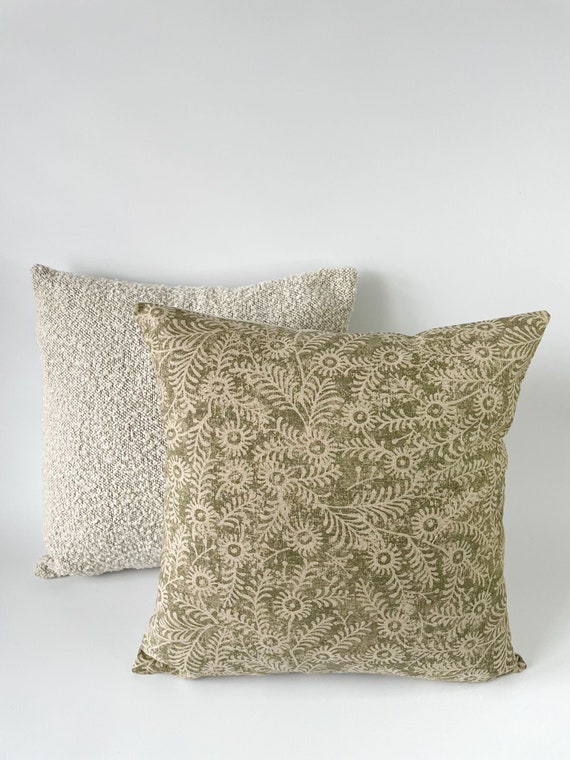This is a vertical color photograph featuring two square, decorative throw pillows positioned against a neutral backdrop. The background is divided into a darker gray upper section, suggesting a wall, and a lighter gray lower section that seems to be a surface, possibly a counter or floor. The pillows cast subtle shadows onto the surface behind them, emphasizing their placement.

The pillow in the foreground, located slightly to the right, is predominantly white with a pale olive green hue and is decorated with a detailed pattern of plant leaves or stems in tan. Its design suggests an organic, nature-inspired theme. The pillow in the back, situated to the left and partially obscured, is a muted off-white or dirty ivory color. It has a texturized appearance, resembling the color of vanilla ice cream and suggests a plush, albeit slightly rough texture. Both pillows, with their neutral and nature-inspired tones, appear suitable for placement on an armchair or sofa, adding a touch of subtle elegance to any living space.